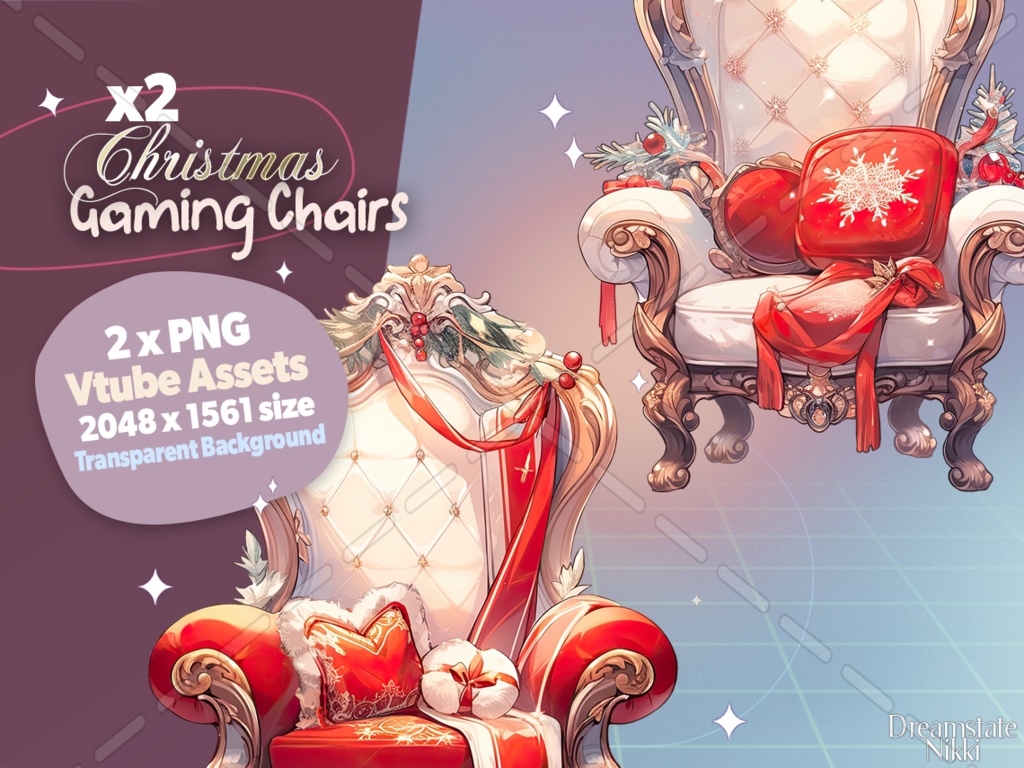This digital rendering showcases two ornate and opulent Christmas-themed gaming chairs. The advertisement on the left side declares "X2 Christmas Gaming Chairs," with the A's stylized with heart shapes in their centers. Beneath this, it notes "2X PNG Vtube Assets, 2048x1561 size, transparent background." Each chair exudes festive Yule-inspired aesthetics, adorned with a rich combination of white and red upholstery accented by holly and mistletoe over the digital designs. They feature high backs and arms with intricate wooden carvings and cushioning that wraps around the wooden base. The pillows are trimmed with fur, some designed to look like presents with ribbons, and one distinct pillow features a snowflake design. A grid-like background is faintly visible, and the chairs, though partly obscured—one with the top and the other with the bottom cut off—are elegantly quilted and draped with red fabric, further embellished with evergreen branches and festive red ornaments.